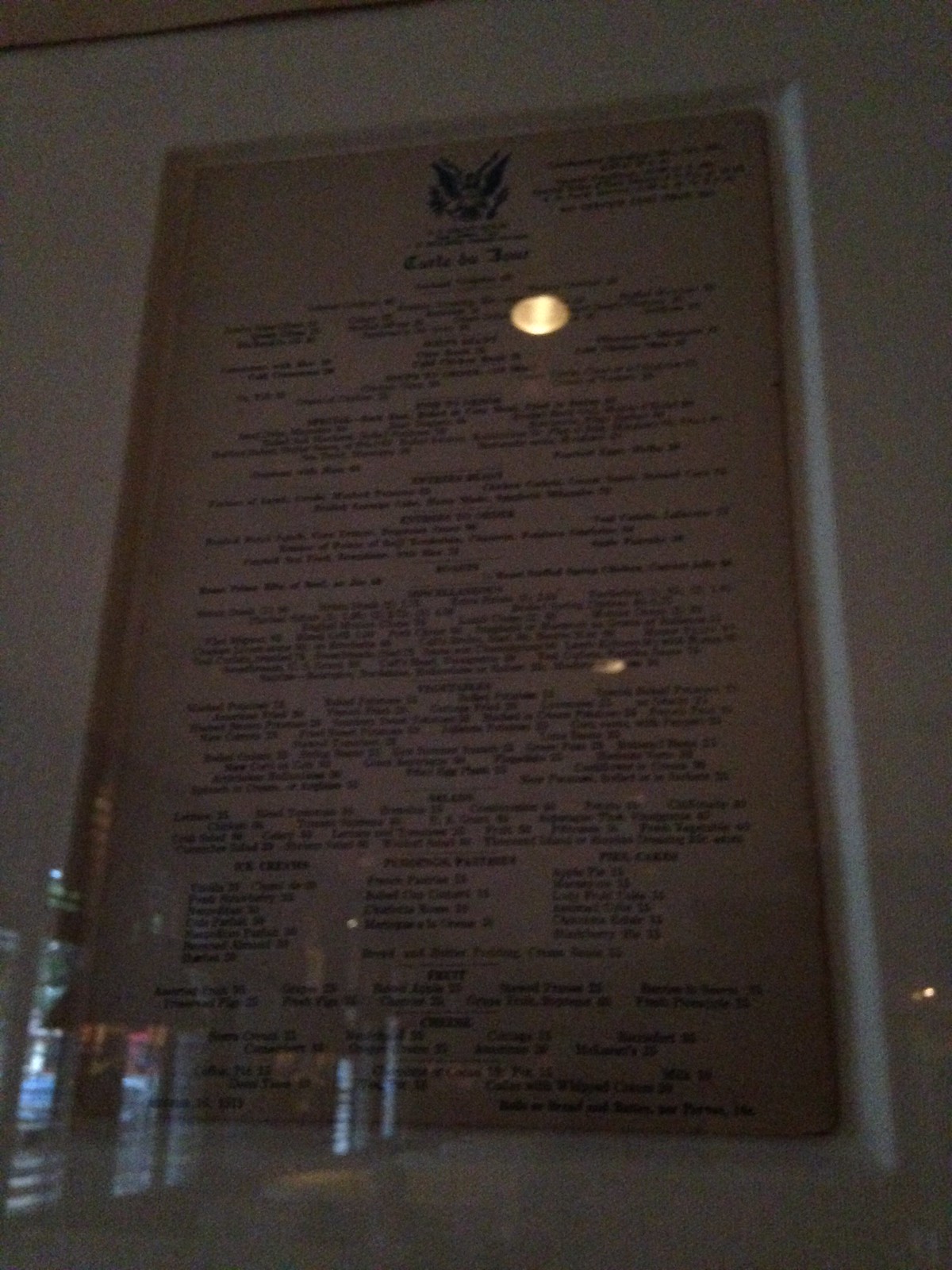This dimly-lit, somewhat blurry photograph captures a vertical-standing menu encased in a white frame, set against a white wall in what appears to be a restaurant. The surface of the framed menu reflects the glow of several light fixtures, adding to the image's haziness. Although the menu's text, written in black, is largely unreadable due to the poor lighting, it suggests a listing of entrees, with what might be drinks listed toward the bottom. The context implies it is situated on a table, though the darkness makes the details difficult to ascertain.